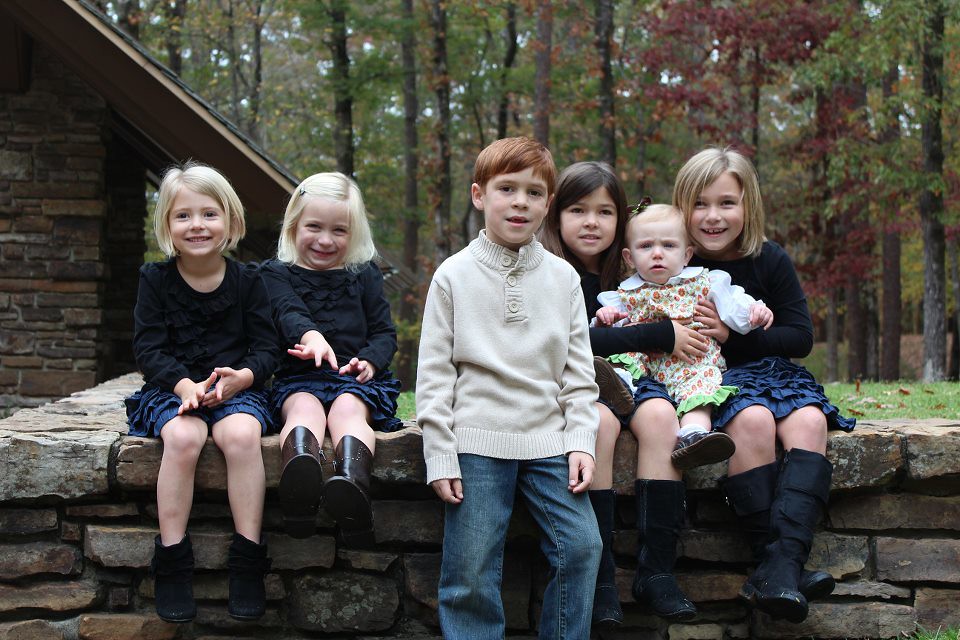This is a horizontal color photograph depicting six children arranged in a line on a gray stone wall. In the foreground, four girls and one boy are positioned on the wall, with the boy standing and leaning against it. The two girls on the far left have light skin, blonde hair, and are dressed in dark blue tops and skirts or shorts, paired with dark shoes. They appear happy, with one girl laughing and the other smiling. The boy in the center has red auburn hair, is dressed in a long-sleeved, cream-colored sweater with three buttons at the neck, and blue jeans. To his right, there's a girl with dark brown hair whose face is just visible behind him, 

Further to the right, another girl with blonde hair wears a blue top and skirt similar to those on the left, along with dark boots. These two girls on the far right are holding a baby on their laps. The baby, with light blond hair, is wearing a white dress adorned with a green and orange pattern, featuring a white collar and long sleeves. The baby has a confused expression while the others are mostly smiling.

In the background, there's the edge of a stone building with a large steep, angled roof to the left, and beyond it, a wooded area with tall, narrow trees showcasing leaves in various shades of green, with some turning red or brown. Small flecks of bluish-gray sky are visible through the tops of the trees. The grass on top of the wall and the dry leaves scattered around add to the autumnal setting of the photo.